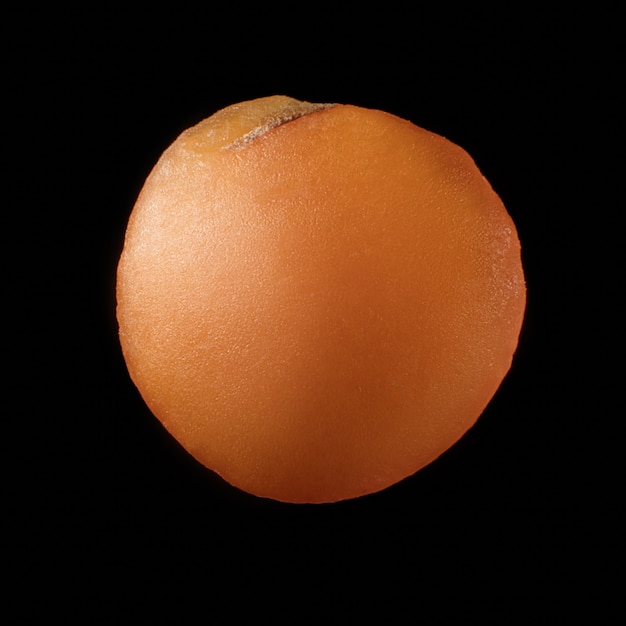This image features a prominent orange fruit set against a completely black background, creating a stark contrast that emphasizes the subject. The orange is nearly perfectly circular although not entirely, with a soft and slightly dimpled texture across its bright orange surface. At the top of the orange, there is a noticeable flat area with a depression, displaying a brownish discoloration that might suggest some damage or imperfection. Additionally, there is a slight yellowing in parts of the orange peel, particularly near the top. The lighting in the photograph is directed from the left, casting a subtle white highlight on that side and producing a shaded gradient on the right, enhancing the three-dimensional appearance of the fruit in this simple, square-shaped composition.